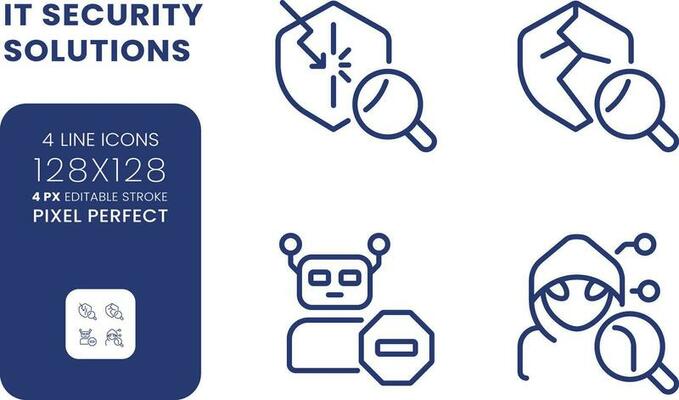This digital image appears to be an advertisement for an IT security solutions company. On the left-hand side, bold navy blue text reads "IT Security Solutions." Below this, a navy blue rectangle contains the following details: "Four Line Icons, 128x128, 4px Editable Stroke, Pixel Perfect." To the right of this text box, there are four enlarged line icons arranged in a two-by-two grid. The top left icon features a five-sided shield with an arrow pointing to the center and a magnifying glass to the lower right. Next to it, the shield is depicted as broken with a lightning bolt through it and a magnifying glass below. On the bottom left, an outline of a robot is shown with a stop sign shape on its lower right. The final icon, positioned to the right of the robot, depicts a hooded figure resembling an alien, with a magnifying glass, symbolizing surveillance or investigation. This sequence of icons visually narrates the progression from standard IT security measures to detecting threats, experiencing breaches, and addressing external control attempts.